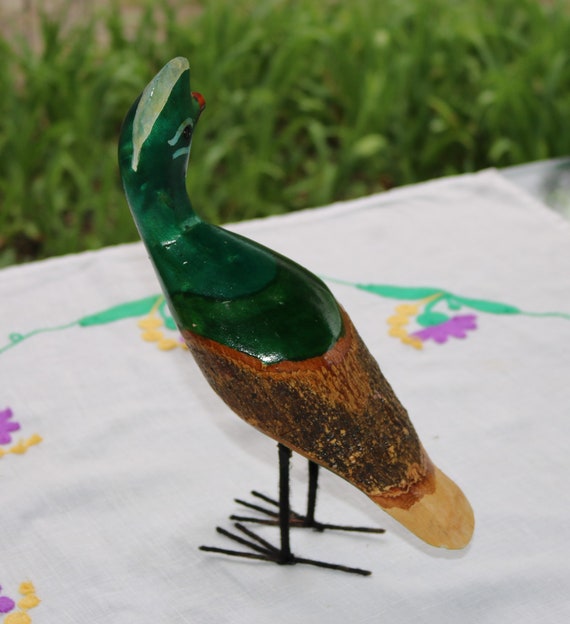This photograph showcases an ornamental bird statue poised on a white tablecloth adorned with an intricate design of purple and yellow embroidered flowers and green leaves. These flowers and leaves form a decorative, minimalist ring around the bird, creating a delicate and cheerful frame. The background is a blur of tall, light and dark green blades of grass, enhancing the natural aesthetic.

The bird itself is carved with meticulous detail. It stands on artificial, black legs, each with three toes. The tail feathers are painted in shades of tan and brown, culminating in a light tan, rounded tip. Moving up from the tail, the bird's body features a blend of dark brown and rust-colored feathers transitioning into a dark green pattern closer to the head. The green of the upper body is interspersed with lighter green accents.

The head is turned slightly, presenting a side profile with a black eye, an orange or red bill, and distinct facial markings. A lighter green or gray line runs down the center of the head, flanked by a straight line below the eye and a curved line above it. The avian ornament, with its vibrant colors and textured appearance, is a striking centerpiece against the white tablecloth and the lush greenery in the background.